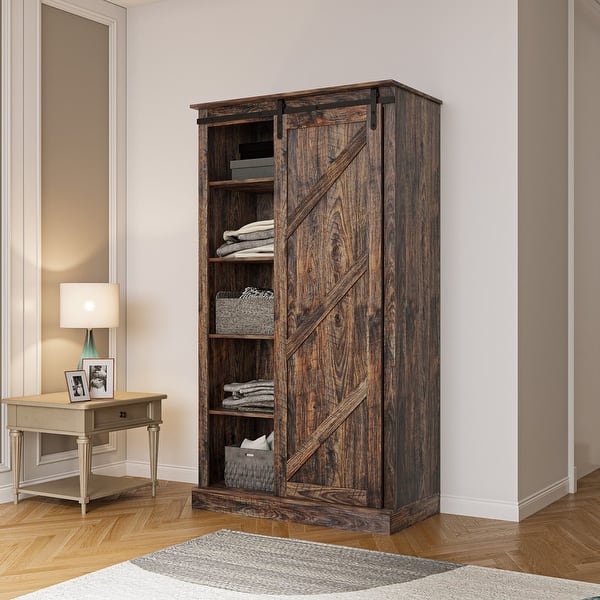The image displays a living room with white walls and a wooden floor. At the center of the room, there is a prominent brown wooden storage cabinet featuring five levels, with its left side open for visibility. The cabinet houses various items: a black and grey box on the top level, white and grey blankets on the second and fourth levels, and a grey box on the third level. The bottom level contains a grey box holding some white fabric. To the left of the cabinet, there is a small beige square side table, adorned with two picture frames and a white lamp with a green stand. Adjacent to the table, part of the wall appears gray. Additionally, a grey carpet with a dark grey pattern on one corner lies in front of the cabinet. The warm ambient light from the lamp adds a cozy feel to the scene.